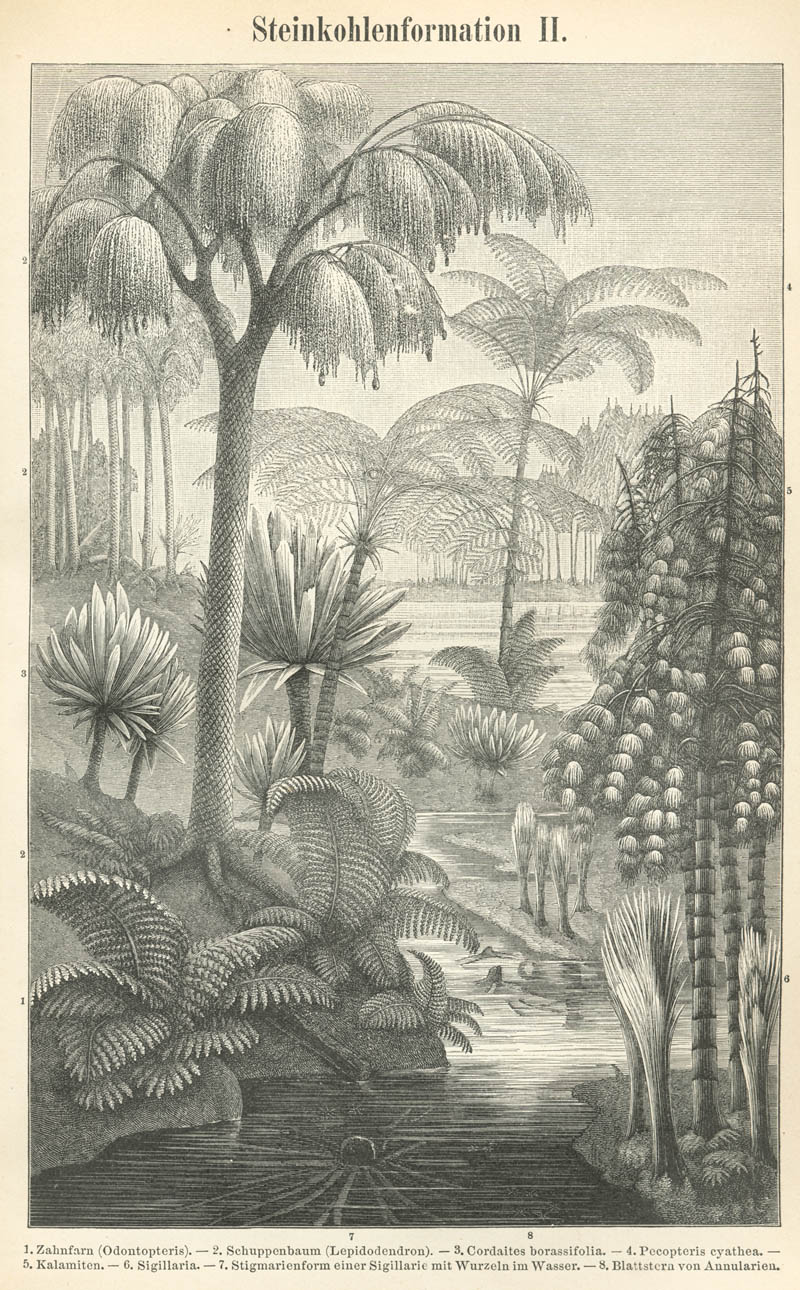This pencil-drawn illustration, appearing to come from a German book, beautifully depicts a tranquil riverway surrounded by diverse vegetations. Prominent throughout the scene are various species of trees, including multiple sizes of palm trees, coconut trees with round fruits, and other distinct flora such as ferns and bamboo. Smaller palm trees line the river's edge, adding intricate detail to the landscape. Annotated numbers dot the image, correlating to a list of botanical names and descriptions in German at the bottom of the page, such as Zahnfarn, Schuppenbaum, and Chorditis Brassifolia. A mysterious black globe-like object can be seen at the center of the river, adding an element of intrigue. The river appears to open up into a larger body of water, possibly a lake, with additional shrubs and a bamboo structure visible along the right-hand side. The top inscription reads "Steinkohlenformation 2," indicating a specific geological or botanical context for this detailed scene. No human presence is depicted, emphasizing the untouched, natural beauty of the area.